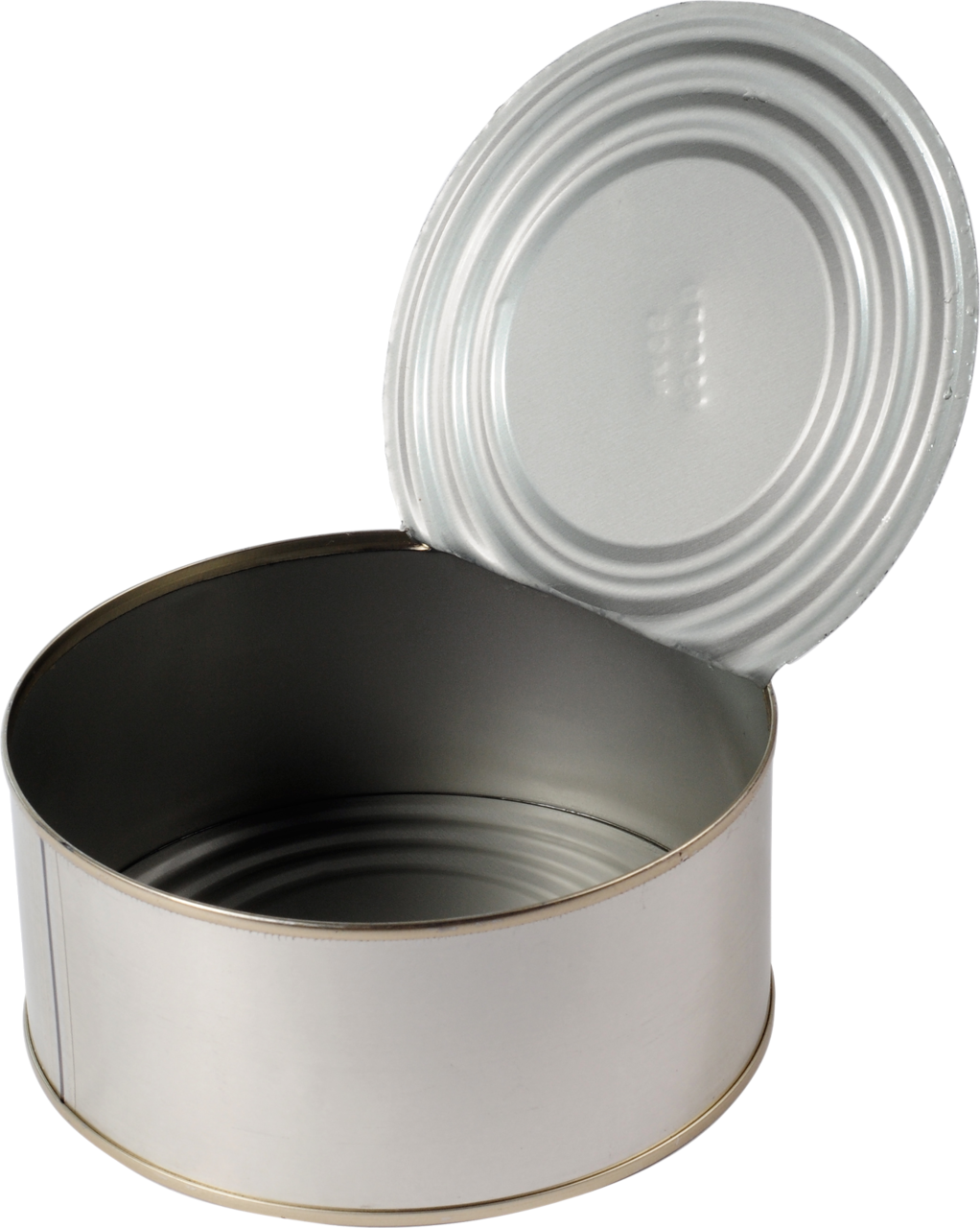This photograph features a small, round aluminum can, reminiscent of a tuna can, set against a completely white background. The can is primarily a lighter silver color, complemented by goldish rings along the top and bottom edges. Its lid has been opened about three-fourths of the way and is propped open, still attached at the right edge. The underside of the lid reveals several concentric circles and imprinted with text and numbers, though they remain unreadable. The can is empty, highlighting its simplistic, template-like design, which is devoid of any labels or specific details, making it appear like a basic, unbranded item. Additionally, there are slight moisture droplets visible on the right edge of the lid, adding a touch of realism to the otherwise minimalistic image.